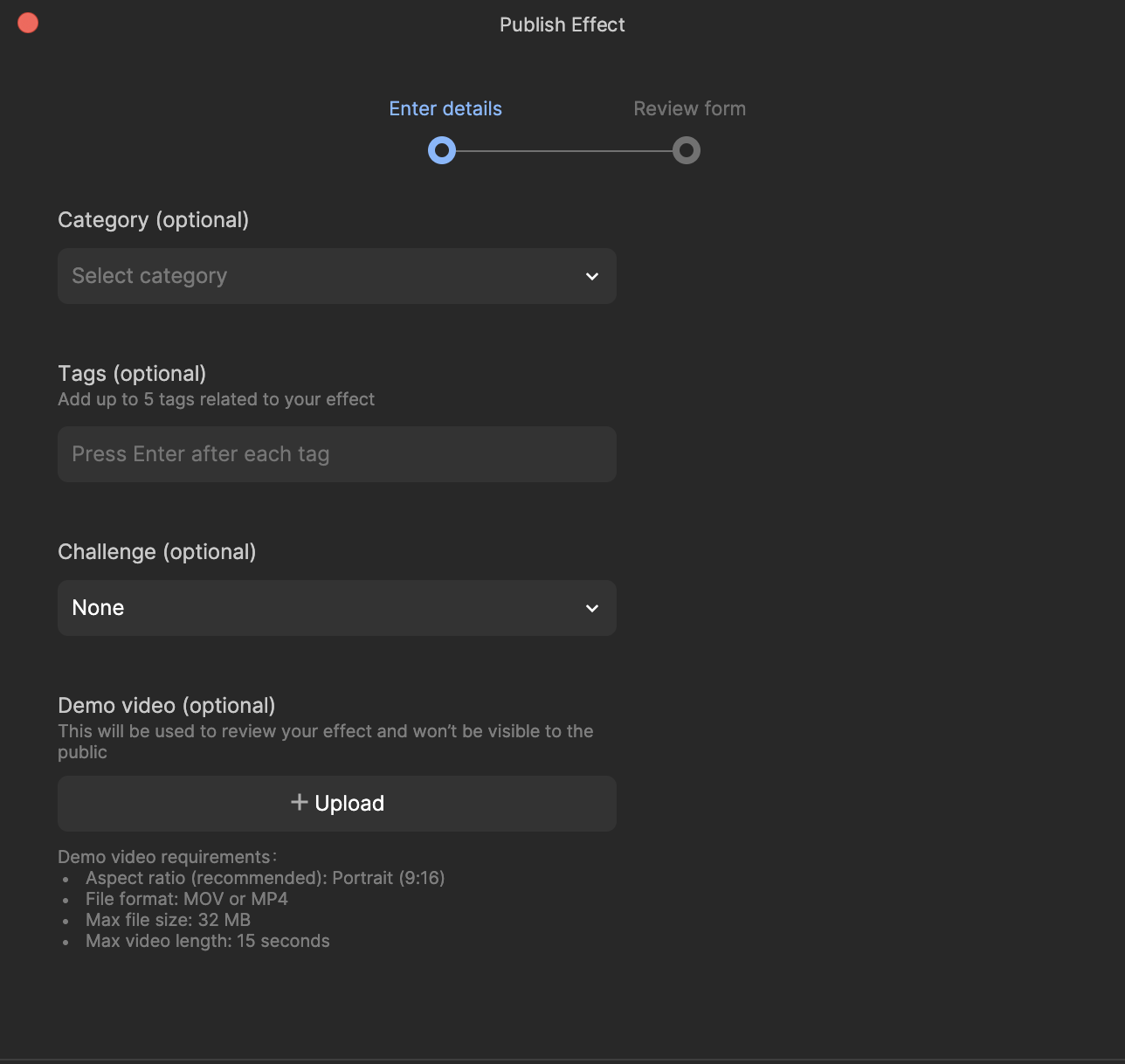The image showcases a "Publish Effect" webpage predominantly set on a black background. In the top left corner, a small red circle features. Central to the header, the text "Publish Effect" is prominently displayed. Beneath this, there is a guiding progress indicator consisting of a horizontal line connected by two dots. The first dot reads "Enter Details" above it, while the second dot indicates "Review Form." The first dot is highlighted in blue, signifying the current step in the process.

Several dropdown menus with headers are visible on the page:
- "Category" which allows the user to select from different categories.
- "Tags" which permits the addition of up to five tags, accompanied by instructions stating to press "Enter" after each tag.
- "Challenge," offering another selection dropdown.

Further down, a section for a "Demo Video" is noted. It is followed by an upload button underneath a header labeled "Button." Text adjacent to the upload button specifies the video requirements, detailing the needed aspect ratio, format, file size, and video length for the demo video.